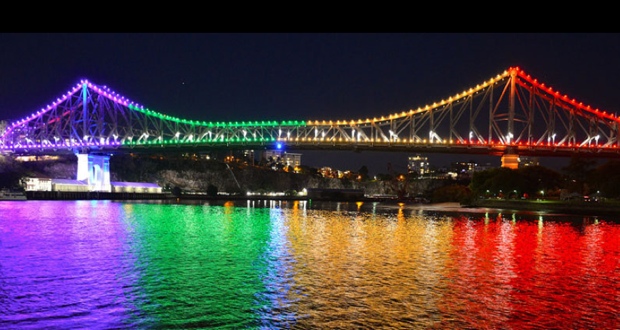This nighttime photograph features a large suspension bridge illuminated in rainbow colors spanning across a tranquil body of water, reflecting an array of vibrant hues. The left side of the bridge is bathed in purple light, transitioning seamlessly through blue, green, yellow, orange, and ending in red on the right. These vivid colors mirror perfectly on the water's surface, creating a stunning visual spectacle. In the backdrop, a cityscape is faintly visible with buildings bathed in soft, normal lighting. Below the bridge and along the water’s edge appears to be a stone seawall or natural cliffs, hard to distinguish in the dark, with a dock running parallel to it and a building situated under the purple section. The sky above is pitch black, highlighting the brilliance of the bridge’s illumination. A solitary black stripe runs across the top of the image, framing this breathtaking scene that could be a nod to gay pride or a similar celebration of diversity.